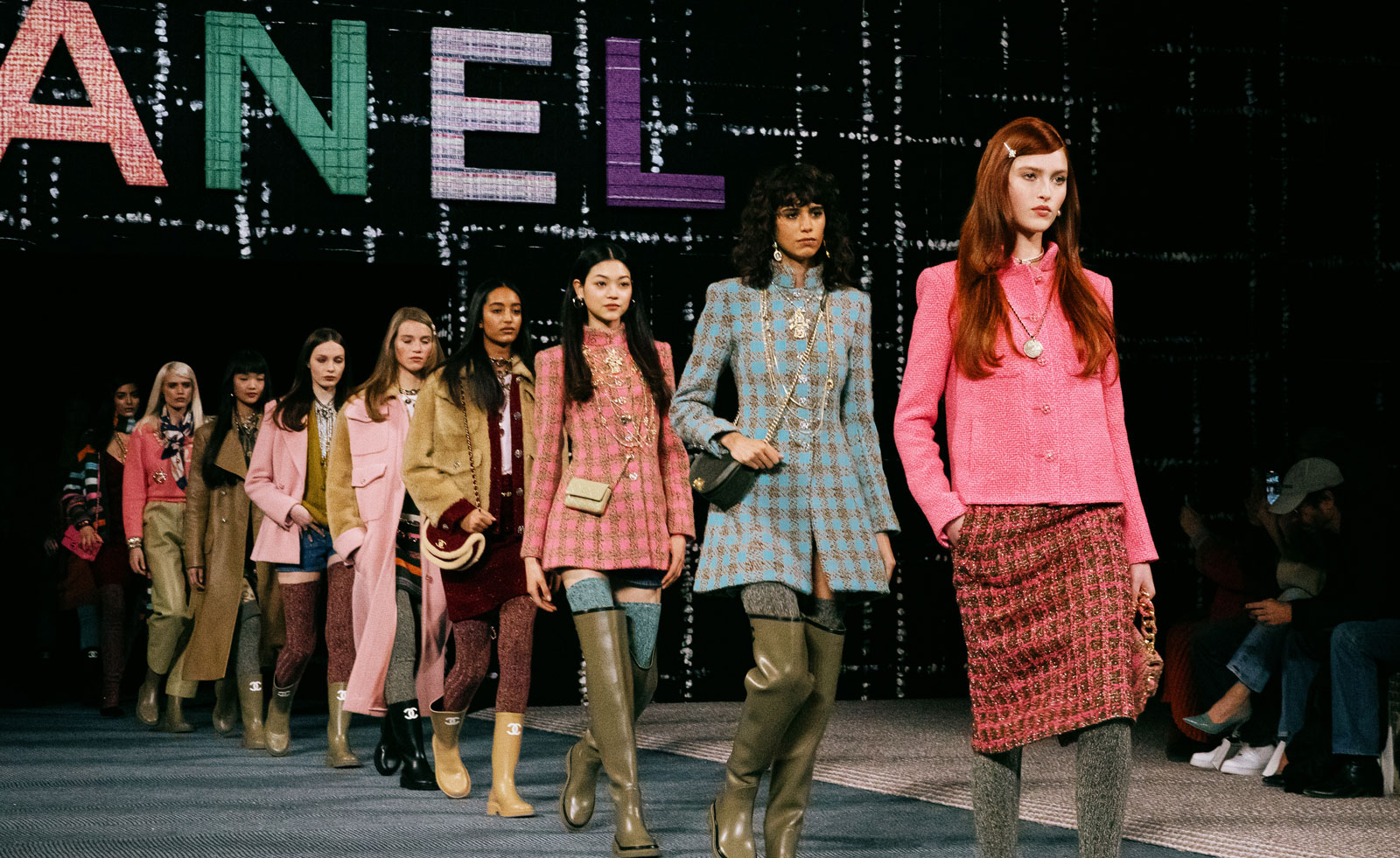In this photograph, a lineup of nine models is captured walking down a runway, suggesting the finale of a fashion show. The runway itself is carpeted in a bluish-gray tone, set against a black background accented with sporadic white dots and vertical lines. Above them, partially visible, is the label "A-N-E-L" in colored lettering: A in red, N in green, E in whitish blue, and L in purple, hinting at the iconic fashion brand Chanel.

The models are donned in vintage-inspired business attire, characterized by bright and autumnal colors—such as the leading model's ensemble featuring a pink jacket and skirt with gray stockings. Their outfits include variations of long jackets, plaid, or flannel prints matched with either stockings, leg warmers, or above-the-knee boots. They carry a solemn and composed demeanor, walking closely together on the runway, which allows only a glimpse of individual details.

On the right side of the image, spectators are visible; three individuals are seated, one notably looking down while wearing a cap. The varied hairstyles of the models—ranging from long red, to curly dark, to long black—complement their different skin tones, adding to the visual richness of the scene.